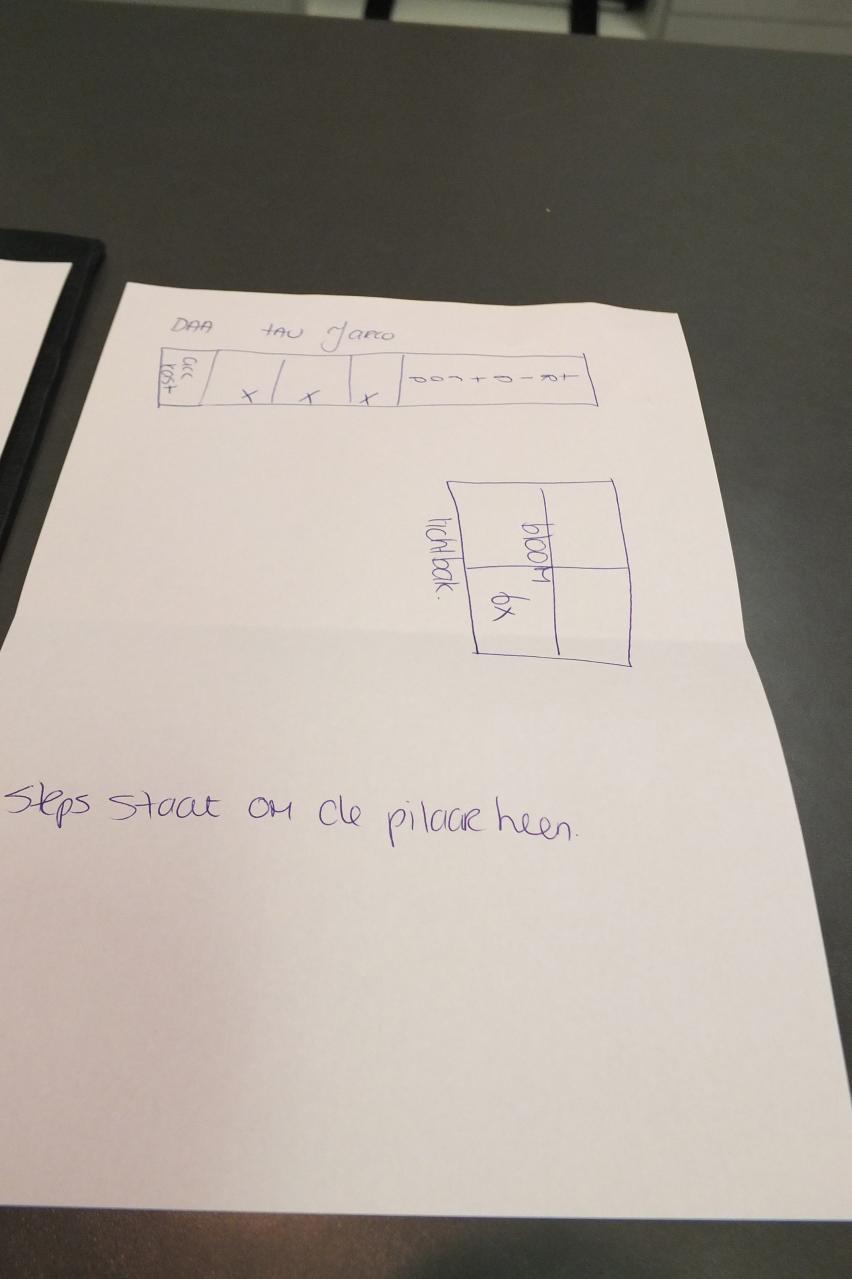This photograph depicts a plain white piece of paper laying on a brown table, next to another white piece of paper of which only the upper right corner is visible. The primary piece of paper appears to have been folded but is now unfolded and shows handwritten text and various diagrams. At the top, in capital letters, it reads "DAN TAR JOMO." Beneath this, there is a rectangular section divided into five sections, containing some illegible lettering and several X marks. Below that, there's another diagram of a square divided into four sections. Towards the bottom of the paper, the text reads, "Steps STAAT OM KLEE PILARHEEN," which seems to be written in a language that resembles English but isn't quite clear. The setting suggests this could be an office, with visible parts of a desk and chair legs on a dark gray floor in the background.